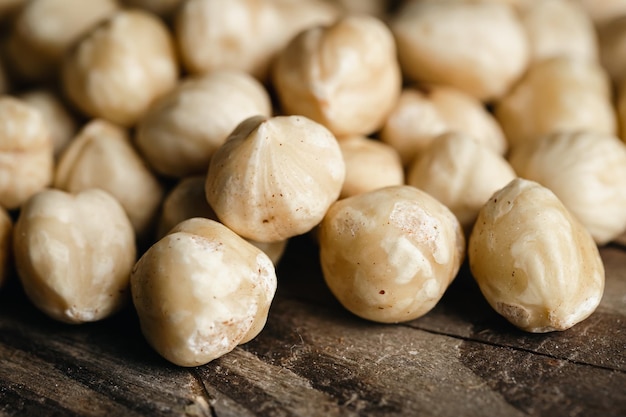This close-up photograph captures a pile of whole hazelnuts spread out on a rustic, wooden table. The table features visible grains and cracks, with a mix of light and dark brown coloring that contributes to its unfinished look. Each hazelnut exhibits a molted tan and white surface with some flecks of black, coming to a point at the tip with lumpy lobes at the top. The nuts vary in focus: those in the foreground are sharp and detailed, while those in the background gently blur out, emphasizing the abundance of the hazelnuts, which take up nearly the entire frame except for the bottom 10% where the textured wooden surface is visible.